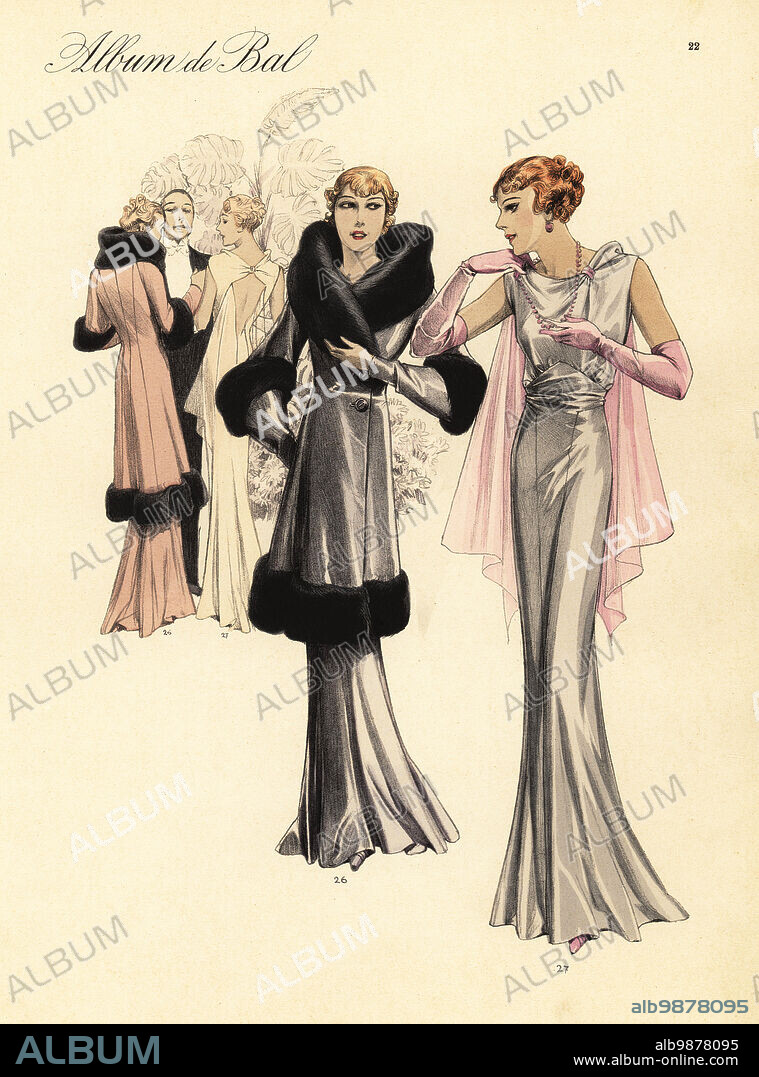The image depicts a vintage-style, hand-drawn illustration reminiscent of the 1920s or 1930s fashion, set against a tan cream-colored background with faint gray and white watermarks spelling "album." The main focus is two elegantly dressed women on the right. The woman on the far right has short orange hair and is wearing a long, flowing silver gown with long pink gloves. She has a delicate light pink cape draped over her shoulders and is holding her right arm close to her neck. Beside her stands a second woman in a similar silver gown, adorned with large, fluffy black fur at the neck, wrists, and hem. Her hand is also raised delicately. Both women's attire appears metallic and luxurious.

In the background, there is a man in a tuxedo engaging with two other women. One woman is in a white dress with blonde hair, while the other, partially obscured, appears to be wearing a peach-colored coat similar in style to the fur-trimmed one but with slightly different coloring. Additional decorative elements include a flora plant, enhancing the vintage ambiance.

At the bottom of the image, there is a black rectangular border displaying the word "album" in blue text. The URL "www.album-online.com" is visible in the bottom right-hand corner, along with "ALB9878095," possibly a reference number. The overall scene suggests a sophisticated fashion illustration, possibly from an old magazine or concept drawing.